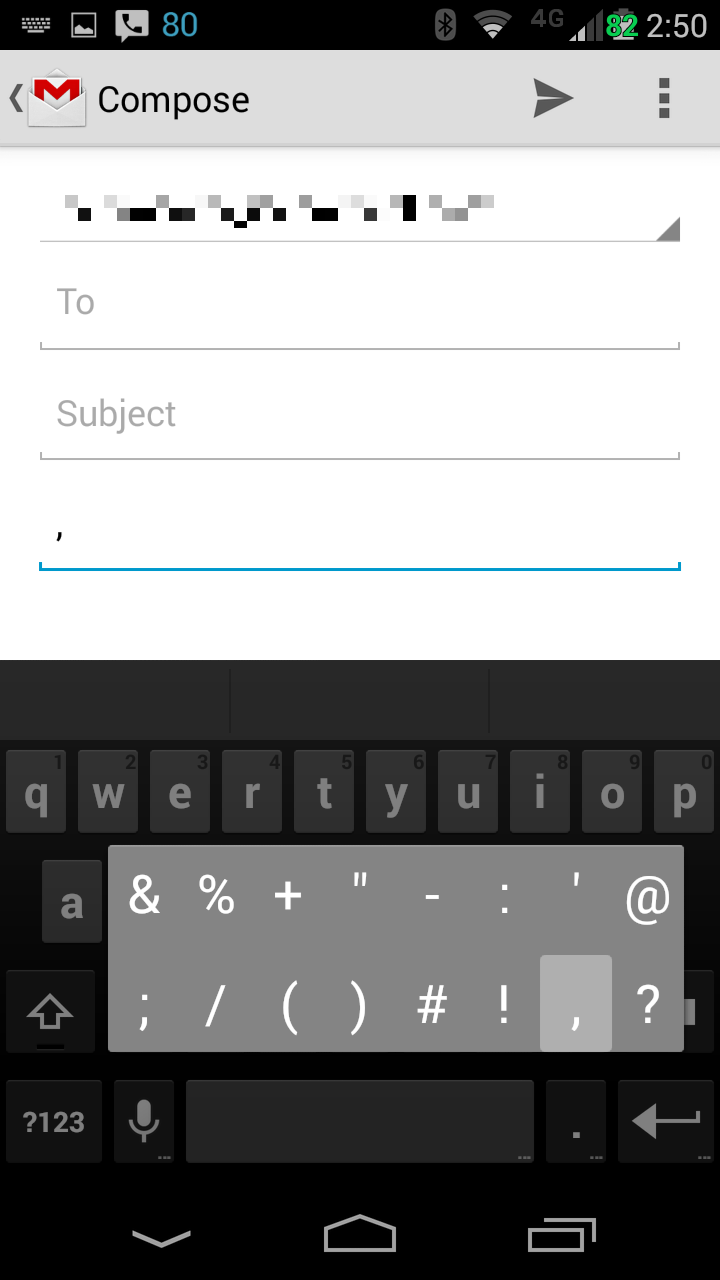This is a detailed screenshot of a mobile phone screen where someone is in the process of composing an email. 

At the very top of the screen, there is a black border. On the left corner of this border is a row of gray icons including a keyboard, photo, and phone call icon. To the right of these icons, in blue, the number "80" is displayed, seemingly representing some form of notification or signal. Moving further right, the number "250" is shown, followed by a battery icon indicating 82% in green. To the right of this battery icon are two full bars of internet signal marked with "4G" next to it, two full bars of Wi-Fi signal, and a Bluetooth icon that appears to be turned off.

Below this top border, the screen background turns gray. On the very top left, there's a dark gray greater-than sign pointing to the left. Next is the email icon, and beside it, "Compose" is displayed in black text. On the far right are three black dots aligned vertically, indicating additional options.

Below this section, there's a pixelated area running across the screen, which seems to contain text. Underneath this area, there's a gray line, followed by the word "To" in gray and a corresponding line underneath it. Below this, it says "Subject" with another gray line underneath it. Further down, there's a blue line indicating the start of the message body.

At the bottom of the screen, the virtual keyboard is visible with a black background at the top and gray keys. The keys are light gray with white letters. The top row of letters includes QWERTYUIOP. On the next line is the letter 'A', which has a popup displaying special characters such as an exclamation point, period, and at sign. This popup has a light gray background with white symbols.

This detailed composition showcases the exact layout and content visible on the phone screen, providing an in-depth look at the email composition interface.